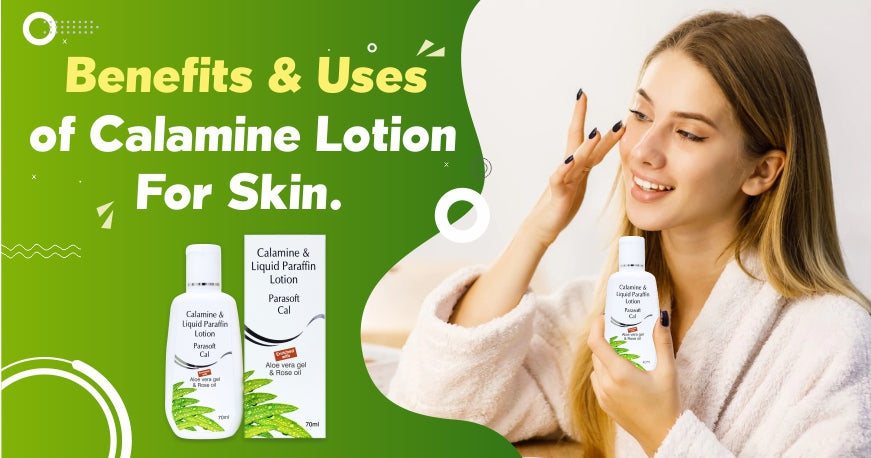This image is a detailed advertisement for Calamine Lotion. The right side of the image features a woman in a white bathrobe, with black fingernails, delicately applying the lotion to her cheek. She holds a bottle prominently labeled "Calamine and Liquid Paraffin Lotion," which also contains aloe vera gel and rose oil. On the left side, the background shifts from green to a yellowish hue, adorned with white circles and semi-circles, adding a visually appealing pop to the image. At the top left, bold yellow text reads "Benefits & Uses," followed by white text stating "of Calamine Lotion for Skin." Below this text, there’s a larger image of the lotion bottle alongside a matching box with the same design and details, including a wavy red and black line and an unreadable red-tilted box. A small image of leaves, likely representing the lotion's natural ingredients, is positioned at the bottom left. The overall layout combines informative text and engaging visuals to effectively highlight the product and its uses.